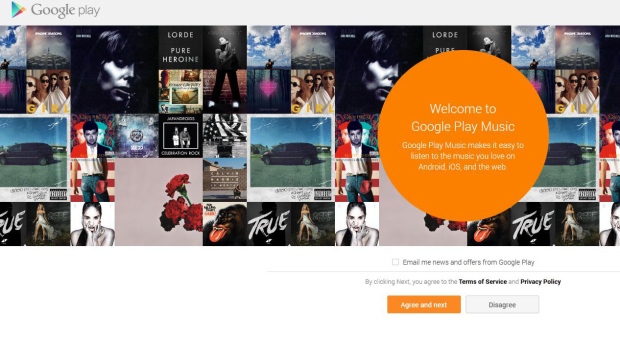In this image, we are looking at a wide horizontal screenshot of a Google Play Music interface. In the upper left corner, there's a gray header with "Google Play" written in dark gray text accompanied by the Google Play icon on its left. 

Below this header, a colorful collage of images is displayed, presumably album covers or artist photos. Prominently at the top, there is an album cover with white text that reads "Lorde, Pure Heroine." The image features a woman leaning against a brick wall, wearing a white hat and looking down. 

Towards the bottom of the image, we see a square with a gray background adorned with three red carnations extending from the right side. Adjacent to this is another square with a slightly blurred depiction of a woman in a long white dress, next to the word "True." 

Dominating the center of the image is a large orange circle with yellow text that says, "Welcome to Google Play Music." Additionally, it explains, "Google Play Music makes it easy to listen to the music you love on Android, iOS, and the web."